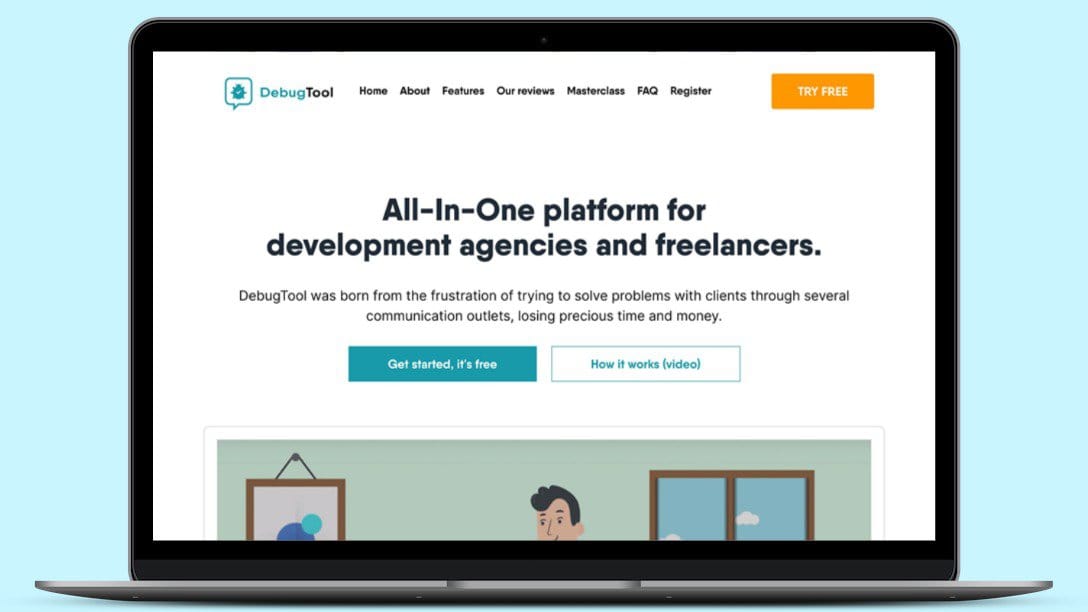The top left corner of the image features a navigation menu with the following options: Debug Tool, Home, About, Features, Reviews, Master Clouds, FAQ, and Register. A prominent orange button labeled "Try Free" is also visible. The main focus of the image centers on a MacBook laptop displaying the text: "All I Want Platform for Development Agencies and Freelancers." 

The tool is described as being created out of frustration from solving client problems, symbolizing the loss of precious time and money. Below the central message, there is a green button labeled "Get Started, It's Free" and a hollowed-out button that says "How It Works (Video)."

Accompanying the text, there is an artistic illustration resembling a painting. This painting includes a blue and green color palette, depicts a scene with a person with hair, a window with a blue landscape, and a nail hung frame. The edges of the window are brown, and the surroundings of the monitor are white with a black border and a silver casing.